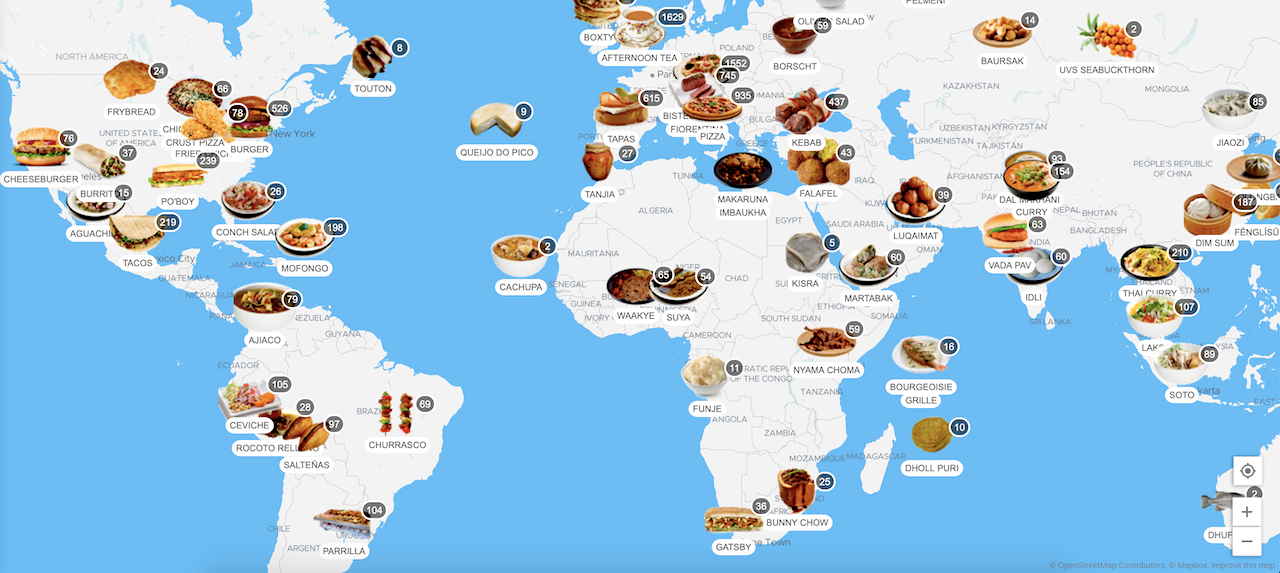The image depicts a detailed, horizontally rectangular, full-color interactive map of the world, devoid of any border, with a bright blue background. Various countries and continents, including North America, South America, Europe, Asia, Africa, and Australia, are illustrated in white and labeled in blue. Scattered across this map are full-color photographs of popular local foods, each labeled with a number and a description. Examples from the United States include dishes like cheeseburgers in the northwest, fried chicken, various burgers, and po'boys in Louisiana; specific foods such as fry bread associated with Native American culture are also visible. Across the world, prominent dishes are illustrated such as tacos and pizzas in Italy, shish kebabs in South America, various soups in Scandinavia, rice and noodle dishes in Asia, and fish near Perth, Australia. The map is designed as a taste exploration guide, though the small, compressed text may be difficult to read. In the lower right-hand corner, there is a plus or minus sign for zooming in and out to view the detailed content better.